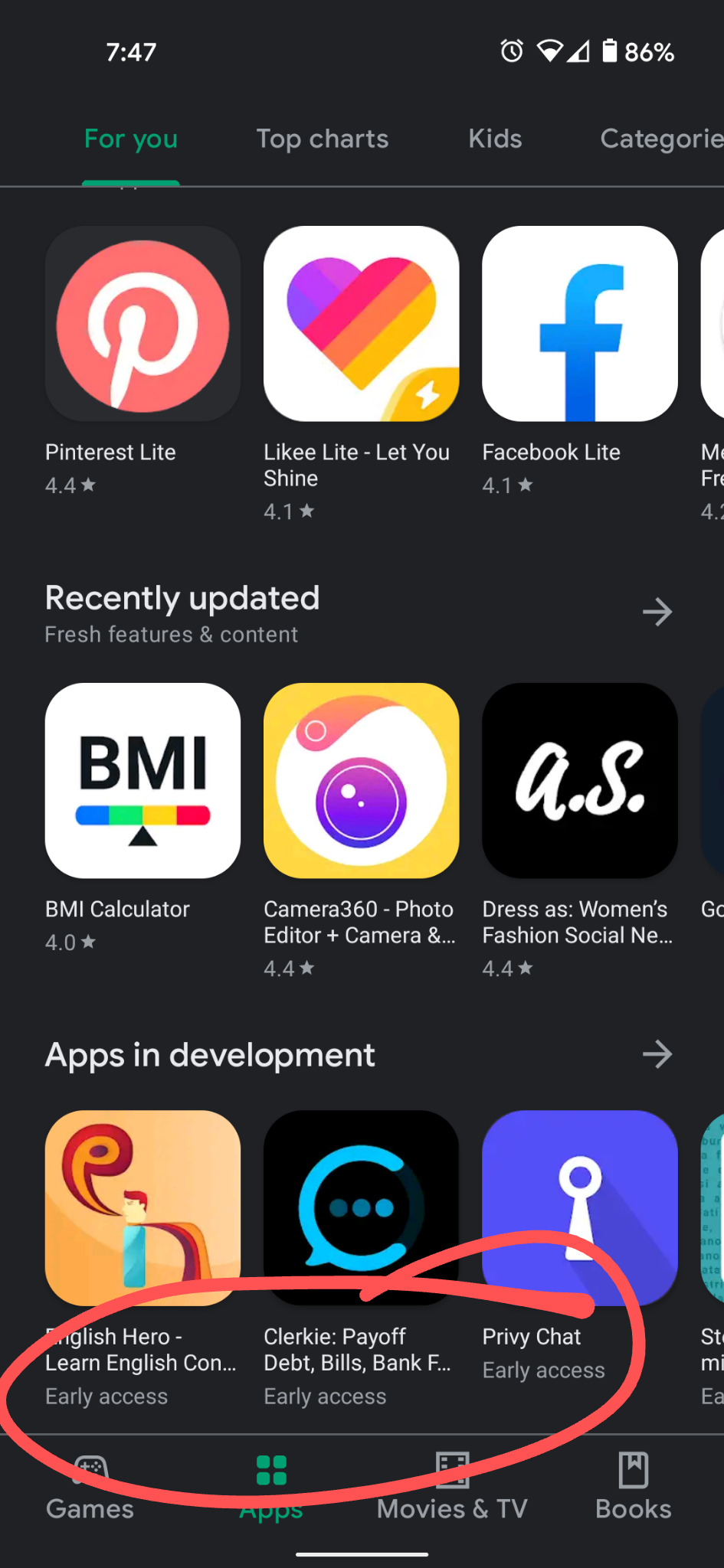The image has a black background and features a screenshot from a phone. The phone screen shows the time as 7:47, the battery level at 86%, and about half of the signal bars are visible. 

The main section of the screen displays a "For You" tab highlighted in green, with a green underline, under the "Top Chart" and "Kids" categories. 

The "For You" section showcases various apps with the first app on the left being Pinterest, identifiable by its red oval logo with a white "P" in the center. To the right of Pinterest is a white box with diagonal rainbow stripes and a heart; it is labeled "A Lanky Light - Let You Shine."

Further to the right is the Facebook Lite icon, indicating the app "Facebook Lite."

At the bottom of the screen, another section labeled "Apps in Development" shows three icons with respective app names: "English Hero - Learn English," "Clerky - Pay off Debt Bills Bank Easily," and "Privy Chat - Early Access." The final app, "Privy Chat," has been circled in red.

The overall layout of the phone screen provides an organized view of popular and recommended applications.